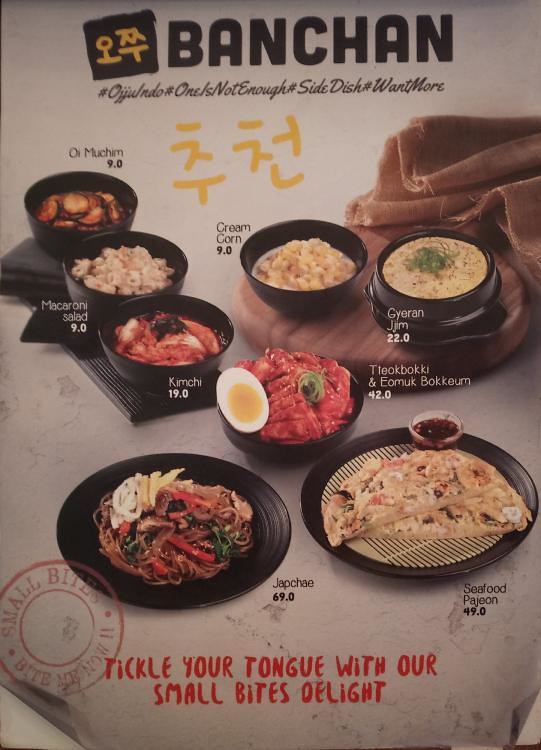The image is a detailed advertisement poster for a Korean food shop or restaurant, prominently featuring a variety of small dishes called banchan. At the top of the poster, in large black letters, is the word "B-A-N-C-H-A-N." Just underneath, there are yellow Korean characters. To the left of the title, within a black rectangular shape, are additional Korean characters. Below the title, several social media hashtags are displayed, which include phrases like "ojundo," "one is not enough," "side dish," and "want more." 

The background of the image is a white or grey gradient, providing a stark contrast to the array of black bowls and plates that hold various dishes, each labeled with their respective names and prices. Some of the dishes include oimuchim and macaroni salad for $9, kimchi for $19, creamed corn for $9, gyeren jjim, tteokbokki, eomuk eokkeum for $42, japchae for $69, and seafood pajeon for $49.

At the bottom of the poster, the tagline "Tickle your tongue with our small bites delight" is written in red, inviting viewers to indulge in the appetizing selection of Korean banchan dishes.